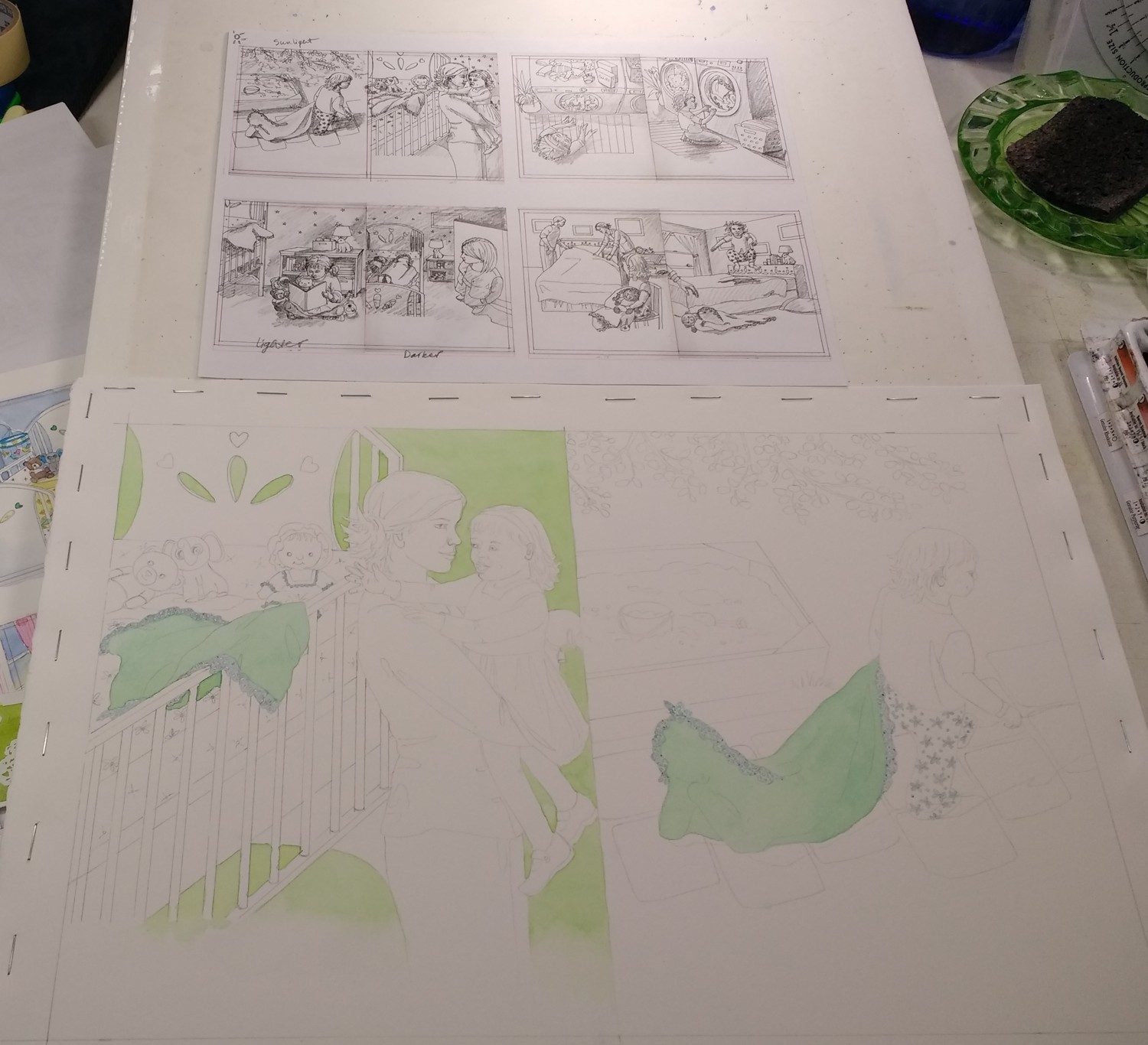The photograph captures an illustrator's workspace, likely on an artist's drafting table. The centerpiece is a hand-drawn series of illustrations that resemble comic panels, each meticulously sketched in pencil. The top part of the image features two rows of cartoon-style thumbnails, telling a tender story of a mother and her child during bedtime. These smaller sketches are juxtaposed with a larger, more detailed watercolor painting that expands on one of the sequences. This larger illustration, stapled to a white glossy background, depicts the mother standing lovingly in her child's bedroom, cradling the child beside a crib with a green blanket. The watercolor in progress only shows hues of green and aqua, emphasizing the background and crib elements. Surrounding the artwork is a tabletop adorned with vintage drawing tools, including a ruffled green glass dish and a pack of drawing implements, possibly brushes or pencils, adding an authentic touch to the artist's creative environment.